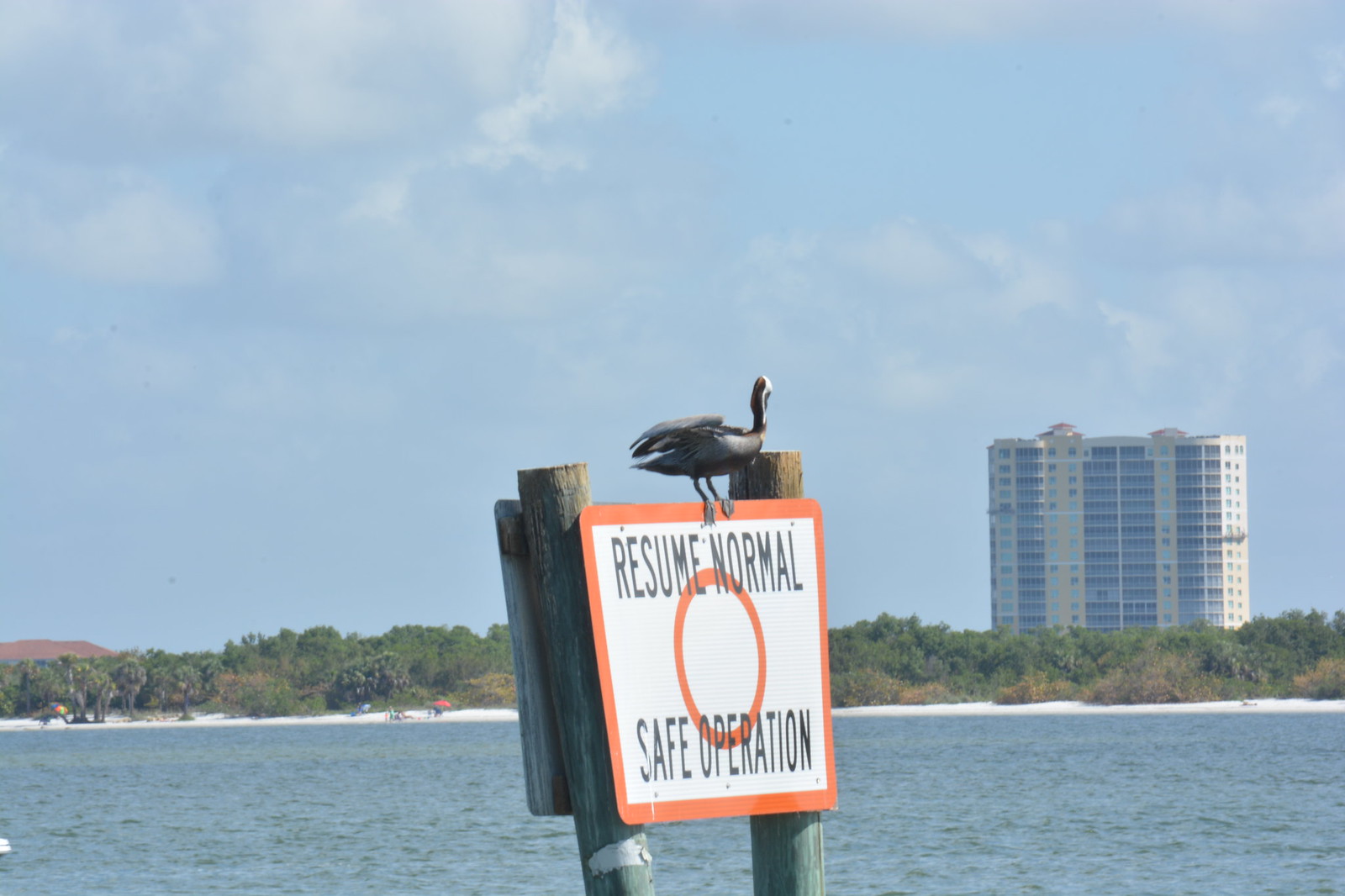This photograph captures a tranquil inland waterway with a diverse and detailed background. In the bottom portion of the image, a serene body of water stretches out, leading to a narrow strip of white sandy beach bordered by lush greenery and a dense array of trees and brush. Just beyond this natural landscape on the left side, a small hill rises gently. Off to the right, a prominent, modern, possibly multi-story white building—potentially a hotel, condo, or office structure—stands against a mostly cloudy sky. This backdrop is slightly broken by patches of blue sky peeking through the clouds. In the middle foreground, a square sign attached to two wooden poles emerges from the water, though the bases of the poles are out of frame. The sign features a red border and a white background with black lettering that reads "Resume Normal" at the top and "Safe Operation" at the bottom, separated by a red circle in the center. At the top of the sign, a bird with gray feathers, a white head, and a black neck is perched, facing right towards the large building in the background. The detailed landscape, with hints of human activity and the crisp, clear message on the sign, provides a peaceful yet dynamic scene likely set in a coastal region such as Florida.